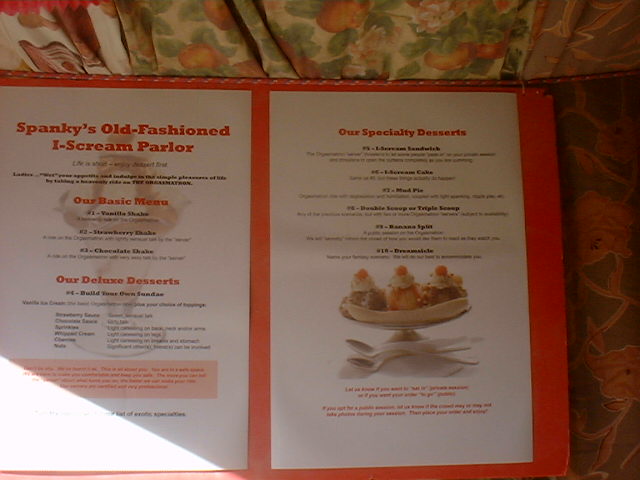The image depicts an open menu from Spanky's Old Fashioned Ice Cream Parlor, with two visible pages. The left page bears the heading "Spanky's Old Fashioned I-S-C-R-E-A-M Parlor." The content on this page is somewhat out of focus, making it difficult to read. However, discernible text includes "Our Basic Menu" with items like "Vanilla Shake," "Strawberry Shake," and "Chocolate Shake" listed beneath it. Below this, there is mention of "Our Deluxe Dessert," though the specific items listed are unclear.

On the right page, the heading reads "Our Specialty Desserts." This section lists various specialty desserts, but the text is blurred and unreadable. Notably, towards the lower part of this page, there is an image of a banana split. The banana split visually features three scoops of ice cream topped with assorted toppings, flanked by a banana on either side. Beneath the bowl of the banana split, there are two white spoons.